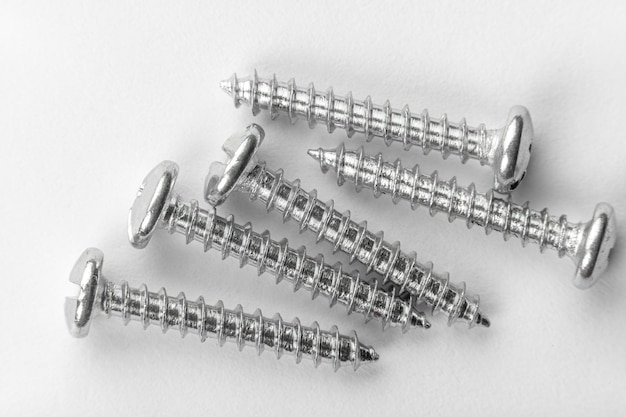The image displays five silver-coated screws arranged against a lightly textured white background. Of these, the two screws at the top have their pointed ends facing left, while the other three screws at the bottom have their pointed ends facing right. Examining the screw heads, it appears that three are Phillips heads and two are Flatheads. The screws dominate the composition, with the heads and shafts clearly visible and neatly placed in close proximity to one another.